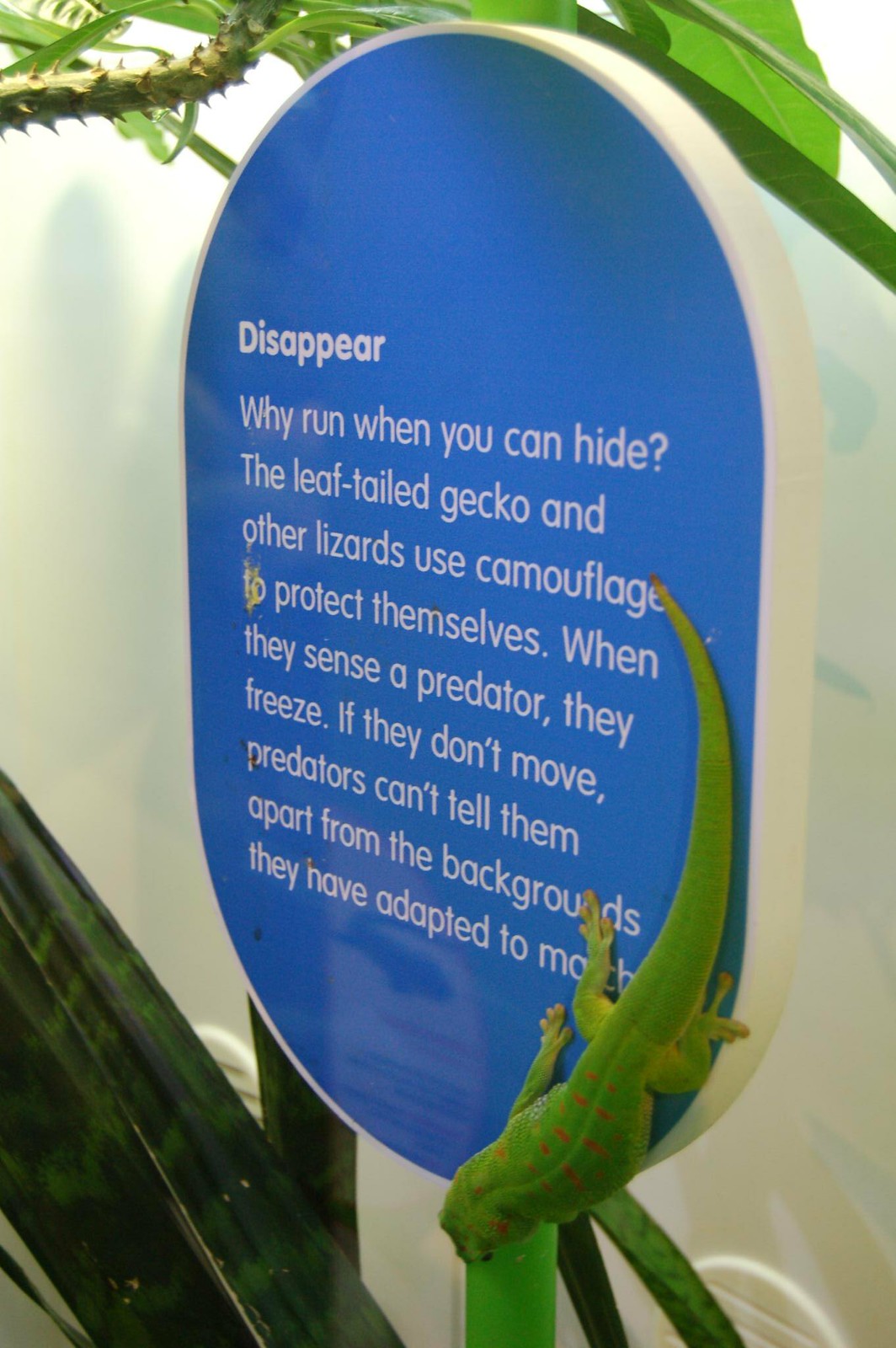In the center of the image, a blue oval sign with white text reads, "Disappear, why run when you can hide? The leaf-tailed gecko and other lizards use camouflage to protect themselves. When they sense a predator, they freeze. If they don't move, predators can't tell them apart from the backgrounds they have adapted to match." To the bottom right of this sign, a bright green lizard with red spots is perched, contrasting starkly against the blue background. The setting appears to be an indoor exhibit, possibly in a zoo, with the top and left edges of the image framed by green leaves resembling palm leaves. The color palette includes shades of green, red, yellow, blue, white, and gray. The sign and the lizard are central to the image, creating a vivid scene that emphasizes the lizard's camouflage capabilities, although humorously, in this case, it stands out against the sign rather than blending in.